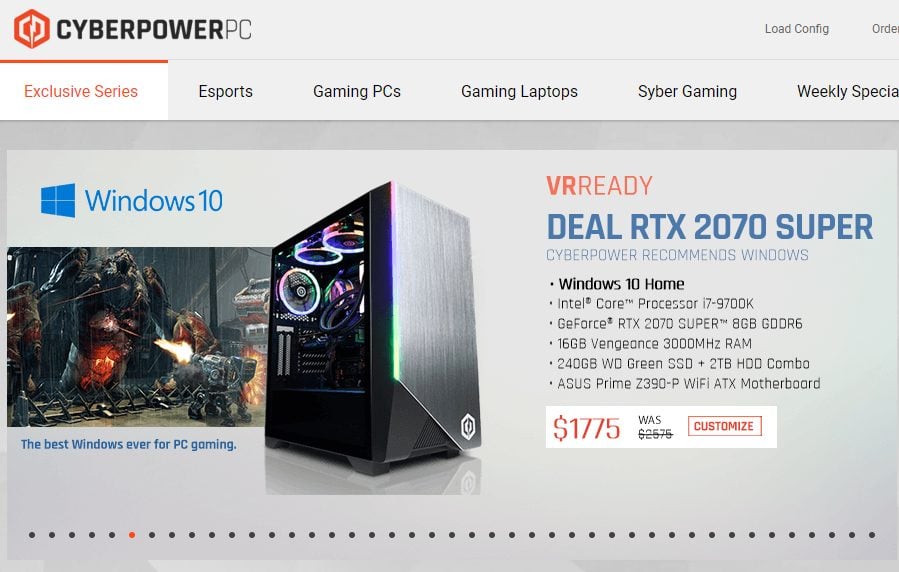This image is a partial screenshot of a website, specifically the upper left corner, featuring a section of CyberPowerPC's homepage. The screenshot highlights two horizontal light gray banners at the top. The first banner contains "CyberPowerPC" with "CyberPower" in bold and "PC" not in bold, alongside the company's icon on the left. On the right side of this banner, in smaller font, partially visible words including "low config" and possibly "order" are displayed.

Below the first banner, the second light gray banner features navigation tabs including "Exclusive Series," "Esports," "Gaming PCs," "Gaming Laptops," "Syber Gaming" (note the alternative spelling with an 'S'), and "Weekly Specials." The "Exclusive Series" tab is currently selected, indicated by its white background and a blue line above it.

Under these navigation banners, the main content shows a featured PC for sale. On the left side of this section, a blue text box announces the system runs on Windows 10, accompanied by a promotional image of a computer game bearing the tagline "The best Windows ever for PC gaming." To the left of this image, there's a detailed photo of the PC tower, showcasing its transparent display case with prominent RGB LED lights.

On the right of the PC image, the product description is presented with key features in orange and blue text. It highlights that the system is "VR Ready" and includes an "RTX 2070 Super" graphics card. Another blue text indicates it is "CyberPower Recommended Windows." Listed below this are the specifications such as "Windows 10 Home," an "Intel Core i7 Processor," a "GeForce video card," memory details, hard drive specifications, and the motherboard type.

The price is prominently displayed, showing a discounted price of $1,759 from the original price of $2,576. Adjacent to the price, a "Customize" button is enclosed within the white box, allowing users to tailor the PC configuration. At the bottom, a series of black dots suggests a slider or carousel feature for browsing through different screens or products.